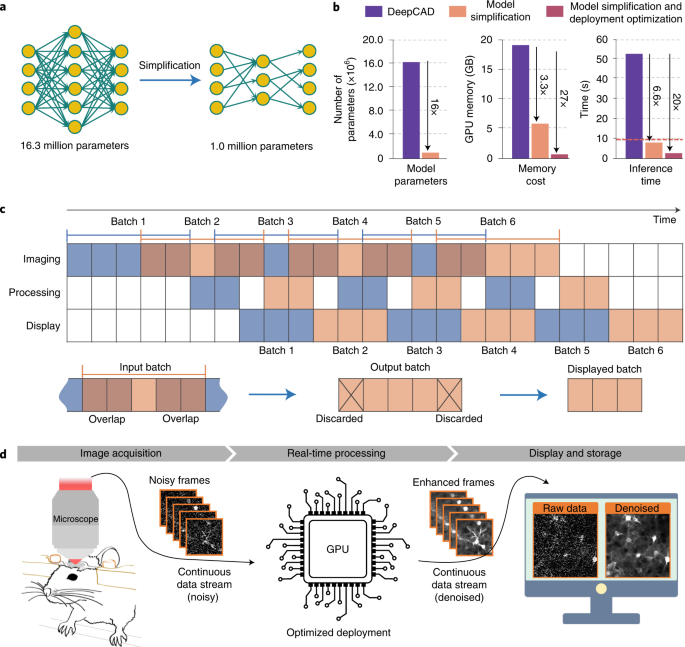The image is a detailed scientific infographic diagram featuring multiple graphs and charts, showing a complex process of data simplification and model optimization. In the upper left corner, marked with "A," the diagram illustrates a comparison of model parameters, starting with a set labeled "16.3 million parameters" connected by yellow circles and green lines, followed by a simplified "1.0 million parameters" representation. Beside this, there is an area detailing "Deep CAD" in purple, "model simplification" in orange, and "model simplification and deployment optimization" in red, indicating various stages and methods applied to the models. 

Central to the infographic, labeled "B," is a set of bar charts comparing model parameters by their reduction across different processes; deep CAD parameters extend considerably compared to those subjected to simplification. 

In the middle section, "C," a sequence depicts batches labeled from 1 to 6, each with detailed steps involving imaging, processing, and display, segmented into colored blocks of blue, orange, and red, as well as some in white.

The bottom section "D" focuses on the entire data workflow: from microscope imaging, acquisition of noisy frames as raw data, to real-time processing on a GPU, resulting in enhanced frames. There's also a mention of continuous data streams and denoising processes. This part includes visual elements such as a mouse under a microscope, a computer chip, and several arrows and boxes illustrating the flow of data.

Overall, the image is densely packed with scientific data and visual aids, intended to convey the intricacies of computational simplification and optimization techniques, likely sourced from an advanced science or engineering publication.